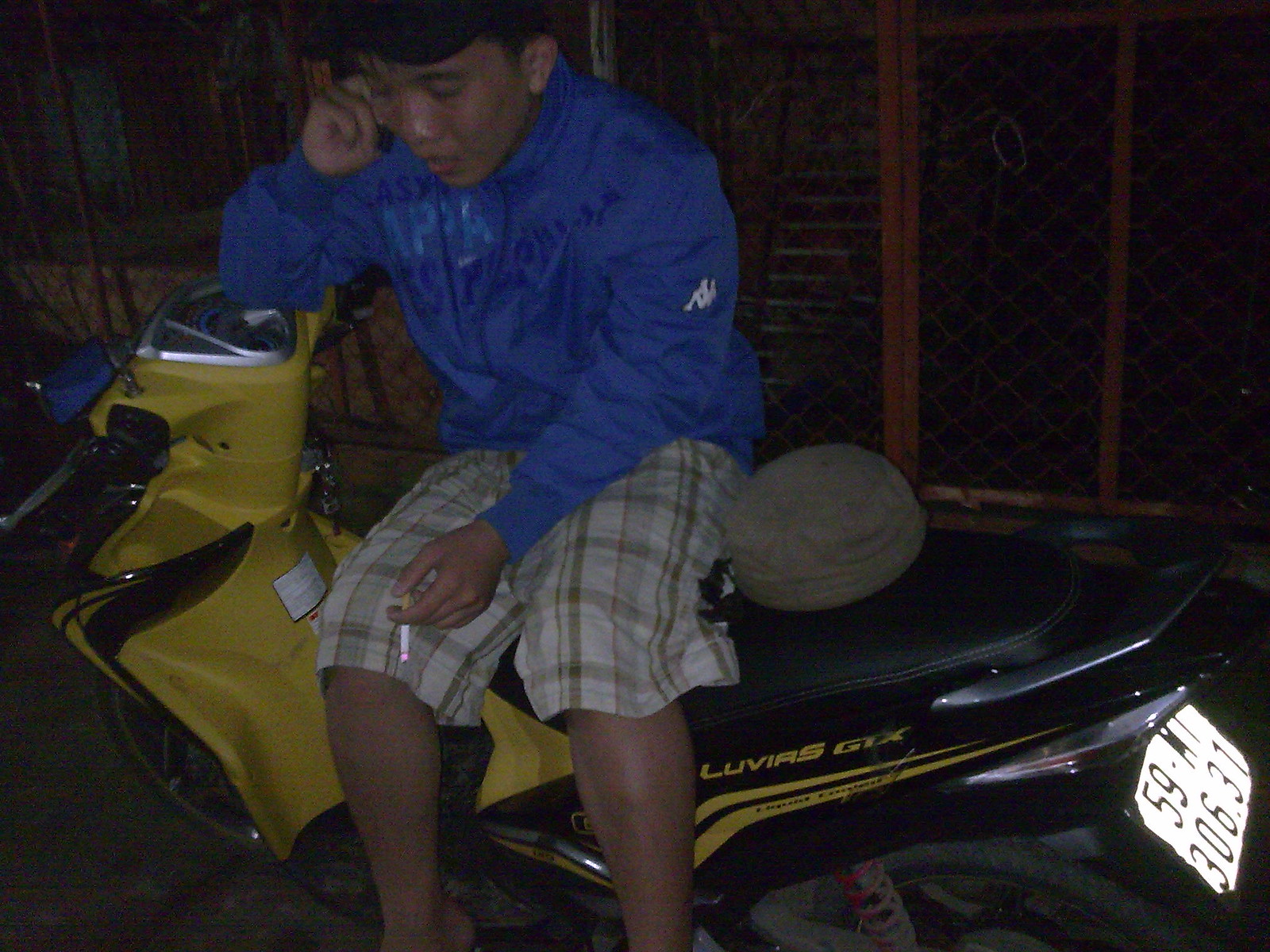A young man, possibly an older boy, is captured sitting on a black and yellow motorcycle, engaged in a phone conversation. The motorcycle prominently features the logo "LUVIR5GTX" in yellow on its rear end. The young man, with black hair, is dressed in a blue jacket and tan plaid shorts. He is seated sideways on the motorcycle, with both legs hanging over the same side, suggesting he isn't preparing to ride it. Next to him, a tan-colored bag or hat is placed. The scene is set against a dark brown background with a building faintly visible, characterized by a distinguishable door. The photograph is overall dark, highlighting the illuminated details, including the license plate on the right rear side of the motorcycle. The subject appears deeply focused on his phone call, not acknowledging the camera.